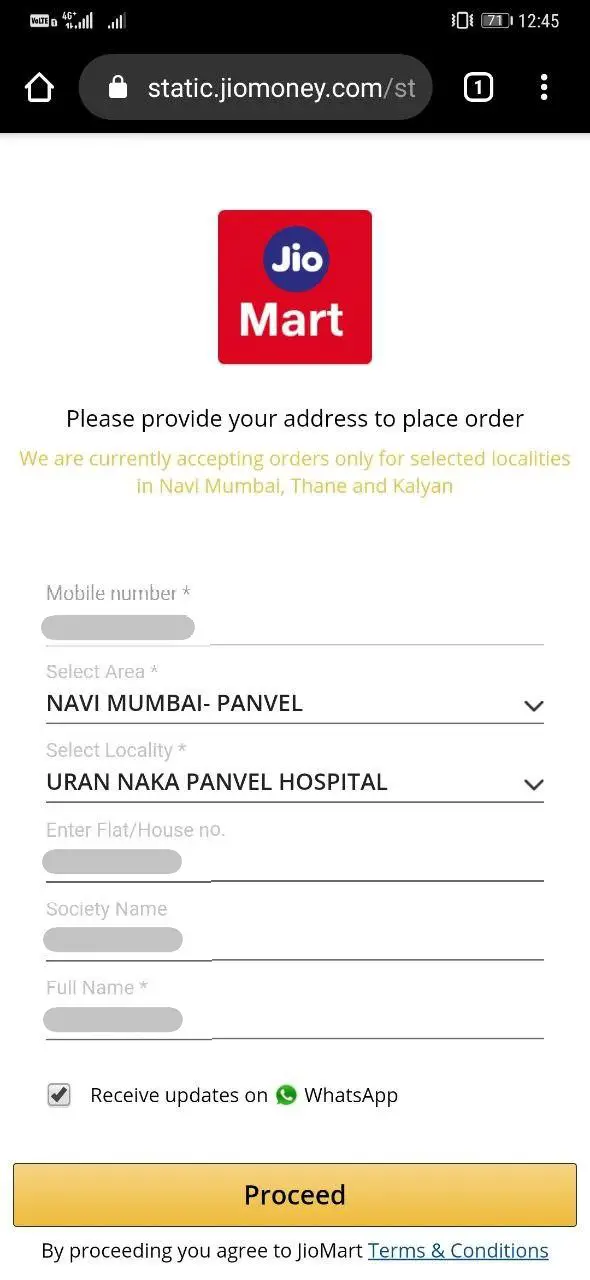Screenshot details displayed on a white background, showcasing a web page from static.jiomoney.com. The interface features the following elements:

- A prominent red square with blue circle containing "G-O" in white text.
- A highlighted message in orange stating: "We are currently accepting orders only for selected localities in Navi Mumbai, Mumbai (spelled out as M-U-M-B-A-I), Thane, and Kalyan."
- A blocked out mobile number displayed in gray.
- Location selection fields including "Selected Area, Navi Mumbai," "Penvale," and "Penvale Hospital."
- User details input fields such as "Enter flat/house number" marked with "N.O." and obscured in gray, "Society name" blocked out in gray, and "Full name" blocked out in gray.
- A check box for receiving updates on WhatsApp, accompanied by a green circle with a white phone icon.
- A prominent yellow rectangle button labeled "Proceed".